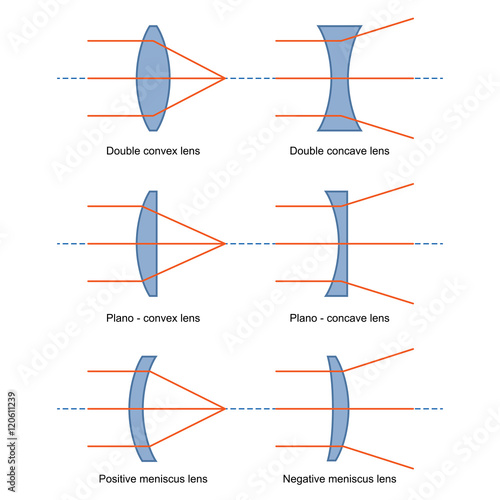This vibrant color infographic, set against a white background, meticulously illustrates the properties of six distinct lens types using blue shapes to depict each lens and orange lines to represent how light traverses through them. Organized in a tall, rectangular layout with three lenses on the left and three on the right, the infographic starts at the top left with a double convex lens, followed by a double concave lens to its right. The middle row features a plano-convex lens on the left and a plano-concave lens on the right. The bottom row showcases a positive meniscus lens on the left and a negative meniscus lens on the right. Each lens illustration includes three orange lines: one passing straight through the center and two skew lines converging at focal points, demonstrating the path of light through different lens shapes. The labeled lenses, designed for educational purposes, assist in understanding light refraction through various lens configurations. Additionally, the Adobe stock number 120611239 is noted in the lower left corner, indicating its source as a stock image.